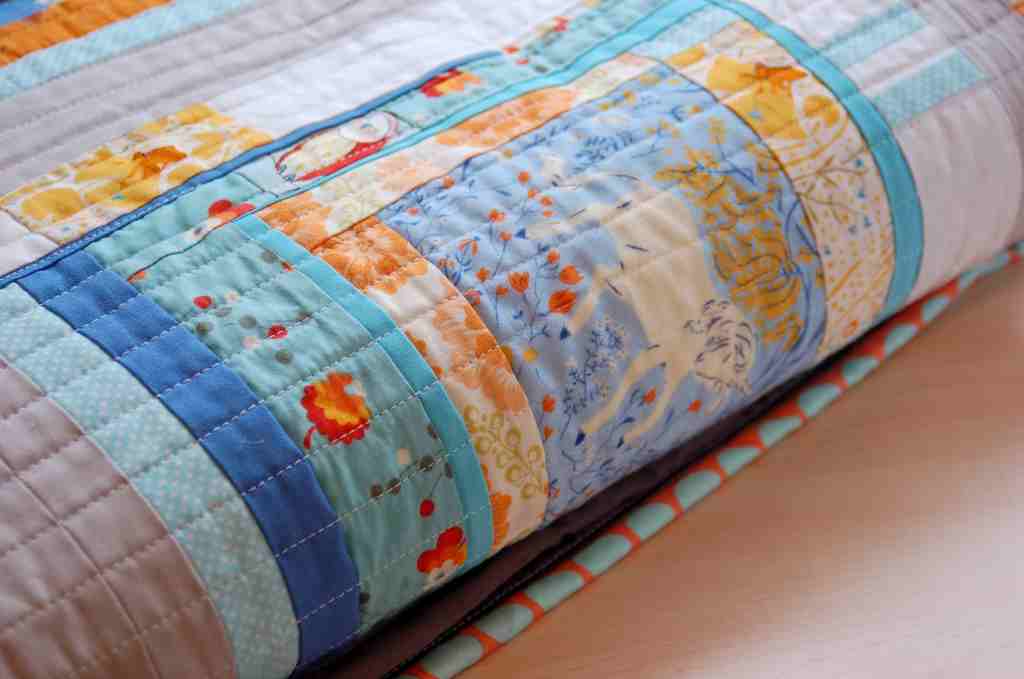This close-up photograph showcases a beautifully detailed quilt resting on a brown surface partially visible in the foreground to the right. Captured at an angle, the quilt's intricate design features a harmonious blend of pale shades including blues, purples, oranges, and pinks, set against a crisp white background. Dominating the composition is a central square showcasing a print with a white animal—likely a horse or unicorn—in a dynamic three-quarter view, cavorting in a meadow adorned with vibrant blue and red flowers. Surrounding this central image, the quilt displays a variety of fabric strips: these include sequences of pinkish-brown, solid blue, light blue or teal with orange flowers, and darker teal blue, punctuated by patterns of orange and brown flowers and leaves. The quilt appears to be machine-stitched, with clear, precise stitching visible throughout, highlighting the meticulous craftsmanship and detailed fabric patterning that evoke a sense of an almost Amish aesthetic.